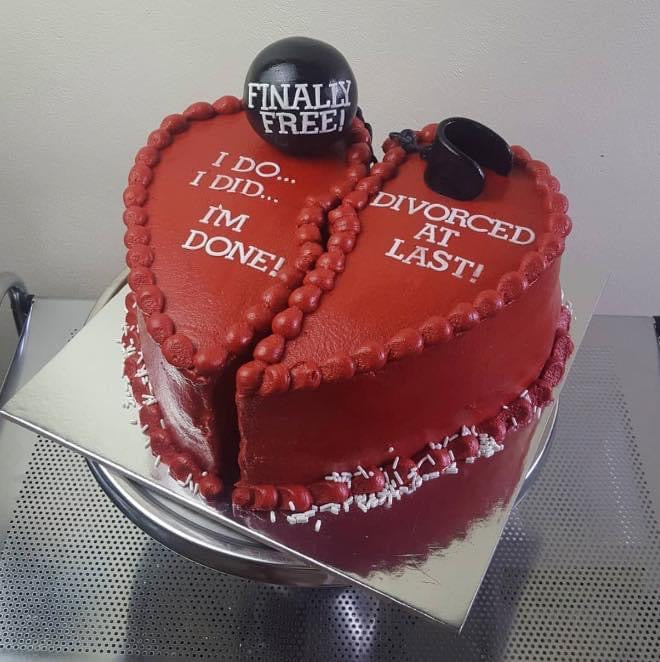This is an image of a "divorce cake," artistically depicted as a broken red heart split into two sections. The cake is adorned with white sprinkles around the base and features poignant messages in white text. On the left side, it reads "I do... I did... I'm done!" while the right side boldly states "Divorced at last!" in all caps. The cake also includes a black ball and chain with the ball labeled "FINALLY FREE!" in all-cap white text, symbolizing liberation. The cake is presented on a square white cake stand with a silver edge, placed atop a rotating round silver base. The entire setup rests on a vented silver tray or counter, with a light gray wall in the background.